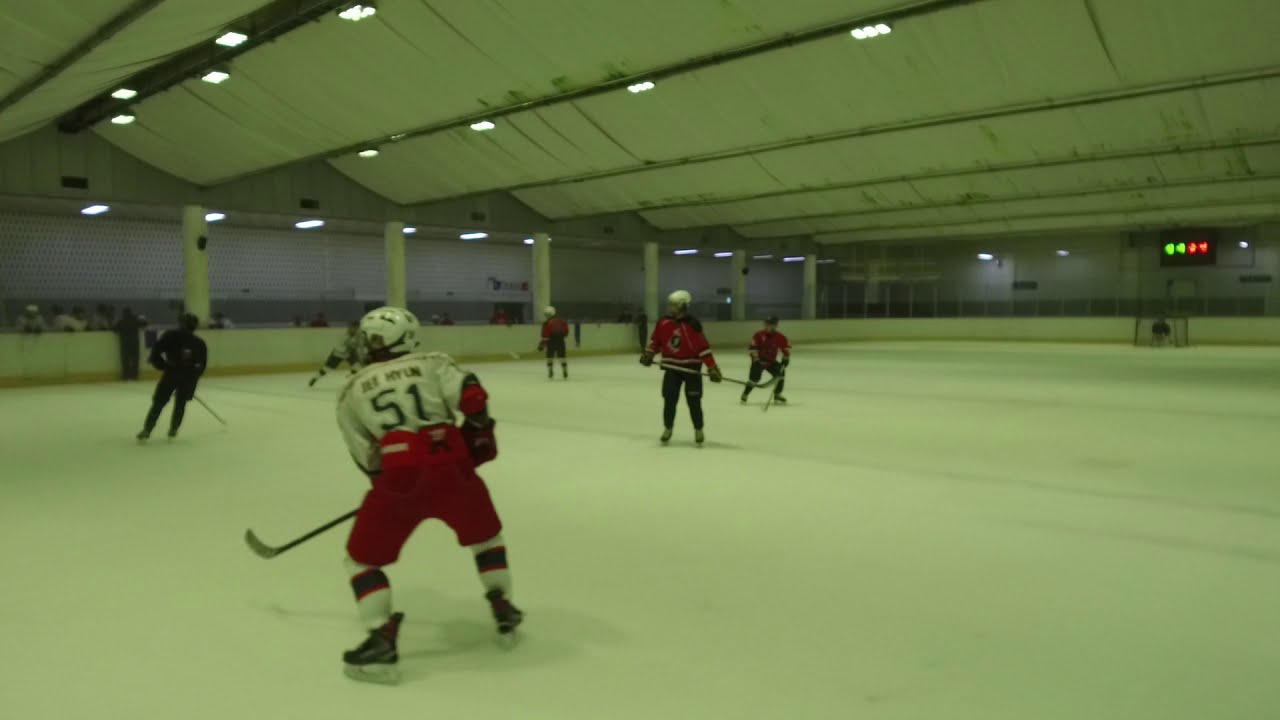The image captures an indoor hockey arena during what appears to be a practice session or non-professional game. The ceiling is characterized by white partitions with a wave-like pattern, illuminated by lights along the higher arcs. On the ice, there are seven visible players: six skaters and a goalie. In the foreground to the left stands player number 51, dressed in a white jersey and red pants, holding his stick to his left. Surrounding him are players in red jerseys and black pants. One player in dark uniform skates towards number 51 from above and to the left, while another in white skates from left to right. To the right of this skater, two players in red face number 51, with one of them holding his stick out. Behind them, another player in red is positioned further back. Distant on the right side of the image, a goalie, in a darker jersey, stands inside the goal, with a scoreboard above him displaying two green and two red dots. The outer wall of the rink has a small group of spectators watching the action unfold.